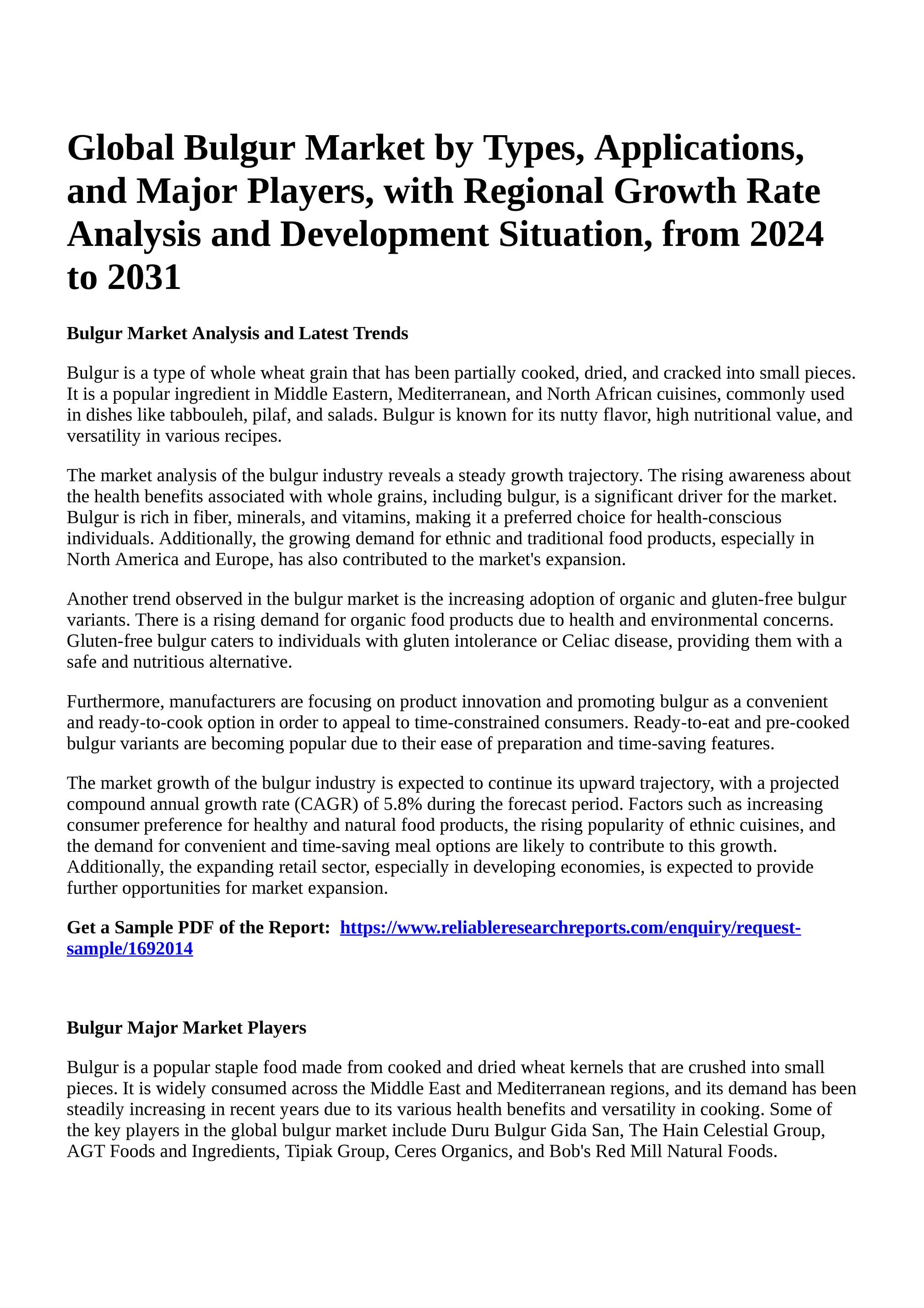This image is a screenshot of a detailed article discussing the global bulgur market. The document, set against a white background with black text, bears the bold header: "Global Bulgur Market by Types, Applications, and Major Players with Regional Growth Rate Analysis and Development Situation from 2024 to 2031." Beneath, a bold but smaller subheading reads, "Bulgur Market Analysis and Latest Trends."

The article is structured into six paragraphs, each consisting of three to six lines of text. The paragraphs analyze the bulgur market, a type of whole wheat grain commonly used in Middle Eastern, Mediterranean, and North African cuisines, discussing its applications and regional growth rate. A bold line, also in smaller font, invites readers to "Get a Sample PDF of the Report," followed by a clickable blue link to a website.

Another section, titled "Bulgur Major Market Players," is followed by a five-line paragraph detailing key players in the market. This comprehensive market analysis seems intended for an audience interested in the latest trends and regional developments in the bulgur market from 2024 through 2031.